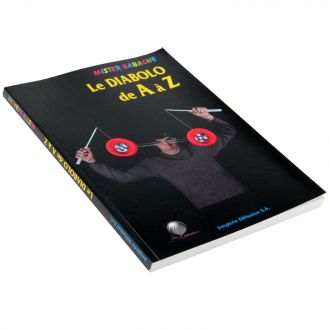The photograph features a black book lying on a white background, tilted slightly counterclockwise to the left. The book's title, "Le Diabolo des," is prominently displayed in yellow font on the upper right corner. Above the title, the author's name, Mr. Babbage, is written in multicolored text that transitions from pink to blue, yellow, and green before repeating. In the center of the book's cover is an image of a man, visible from the stomach up, wearing a long-sleeved, dark-colored shirt. He has black hair and is holding two white sticks in an arc above his head. These sticks are connected by strings to a pair of red wheels with silver centers, which appear to be heavy and pulling the strings downward, creating a distinctive arch.